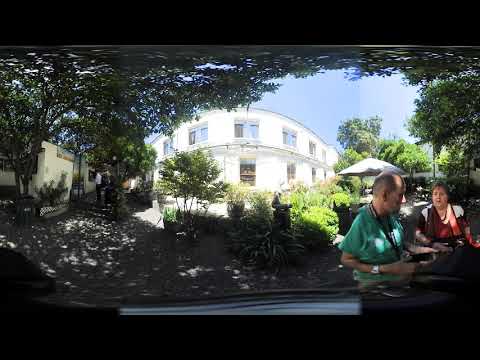This image captures an outdoor scene centered around a beige, two-story curved building with a rounded facade and multiple windows. A clear blue sky and vibrant sunlight suggest a warm, sunny day, with sun rays reflecting off the building. Surrounding the building are lush green trees and bushes that extend to the edges of the photograph, casting ample shade in the bottom portion of the image. In particular, the bottom right corner features an elderly couple, comfortably seated at what appears to be a picnic table or possibly the outdoor section of a restaurant. The man, who is balding, wears a green short-sleeve collared shirt, a wristwatch, and possibly a camera around his neck, while the woman beside him sports a red top and has short hair. Both appear relaxed in the cooler shade, contrasting with the sunlit areas of the image that indicate significant heat. The foreground features brown, sun-dappled ground, adding to the warmth and charm of this scenic moment.